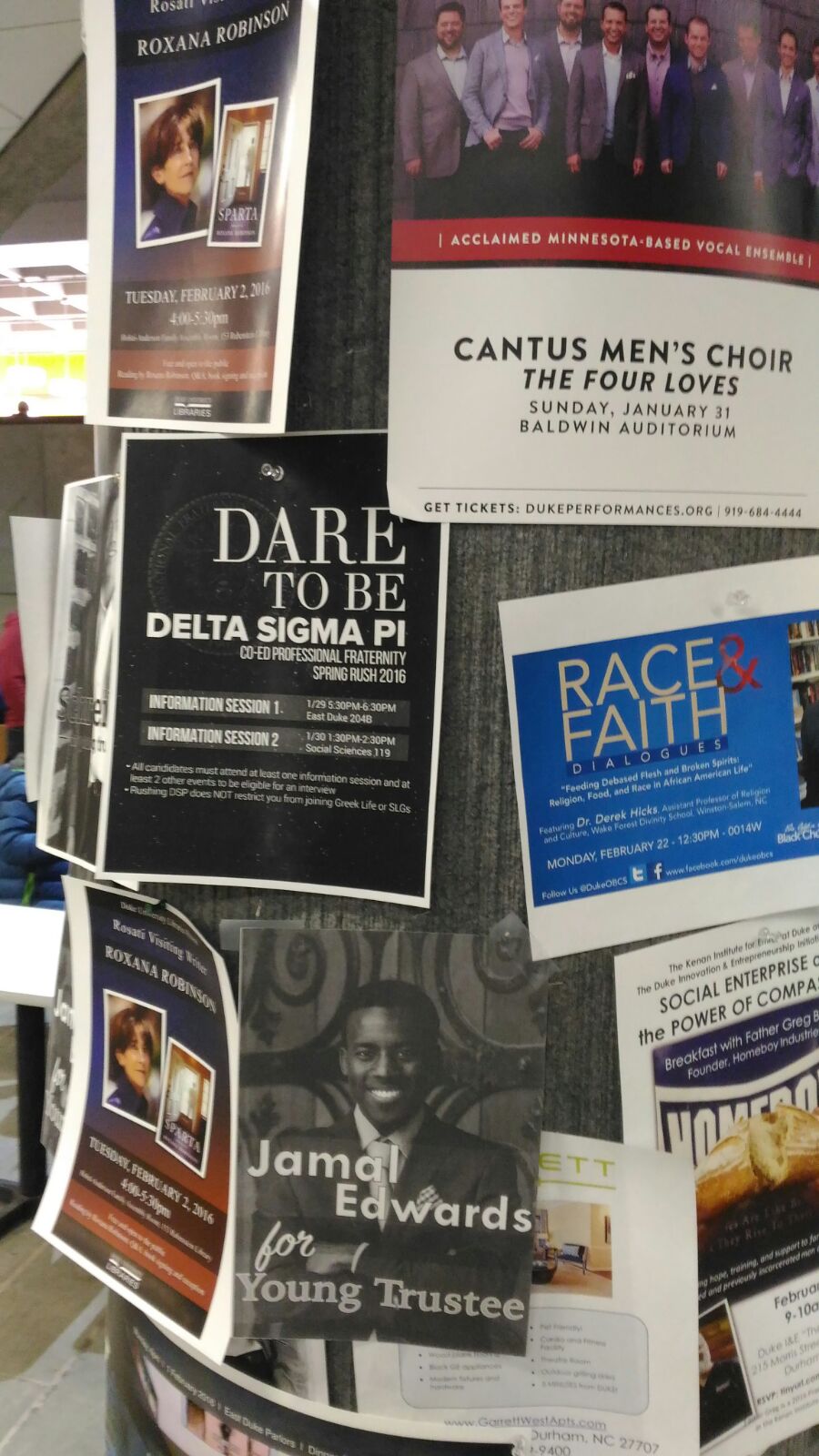This image showcases a streetlight pole with numerous posters and flyers attached, each held by push-pins. The pole itself is gray with vertical ridges running along its length. There are eight distinct posters visible. At the top, a flyer features Roxanna Robinson, a speaker scheduled for a speaking engagement on Tuesday, February 2, 2016. Adjacent to this is a flyer for the Cantus Men's Choir, advertising their performance of "The Four Loves" at Baldwin Auditorium on January 31st, with ticket information provided at Dukeperformances.org. Other notable posters include one for Delta Sigma Pi, a coed professional fraternity promoting their Spring Rush 2016, and another for a Race and Faith Dialogue event on February 22nd. Additionally, there is a black-and-white poster featuring Jamal Edwards running for Young Trustee. The rich array of colors and text styles create a lively, community-focused visual on the utilitarian pole.